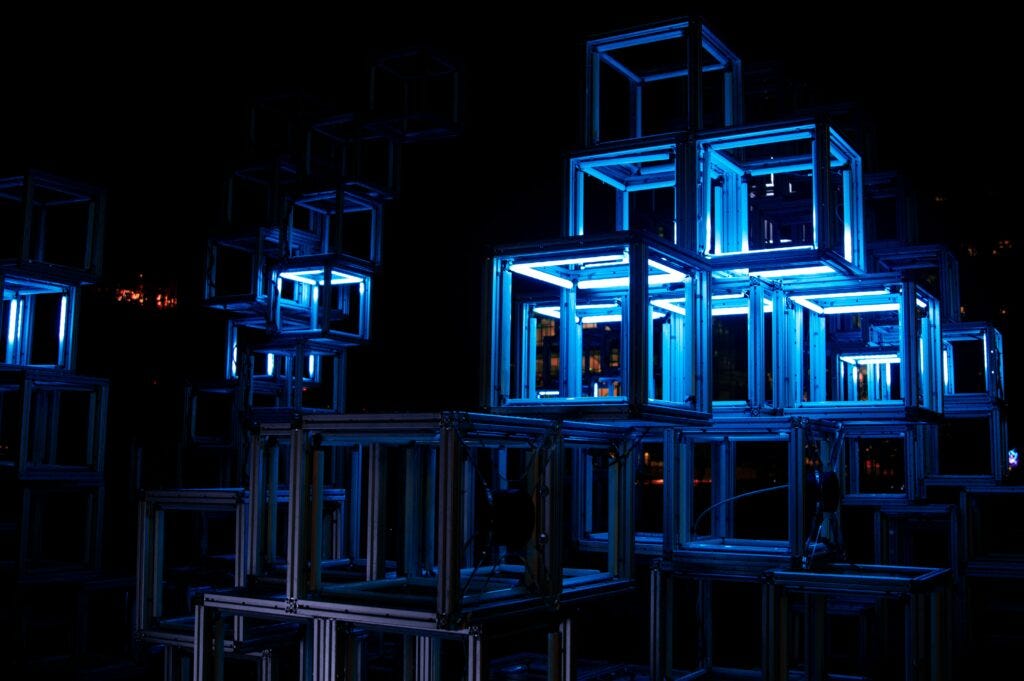In this nighttime image, the dark scene is dominated by a striking art installation comprising numerous stacked metal cubes. Each cube's frame is outlined and illuminated by bright blue LED lights, revealing their transparent structures. The cubes are meticulously arranged, forming a pattern that gives an optical illusion of an obstacle course or a mountainous shape. The top portions of the cubes are predominantly lit, while the lower sections are shadowed. In the background, to the left, a window emits a hint of light as something burns within, adding a subtle glow. To the far right of the image, there are small white dots, and red lights are visible near the bottom, contributing to the overall captivating display. The entire scene is set against a pitch-black backdrop, emphasizing the luminous and geometric beauty of the cubes.